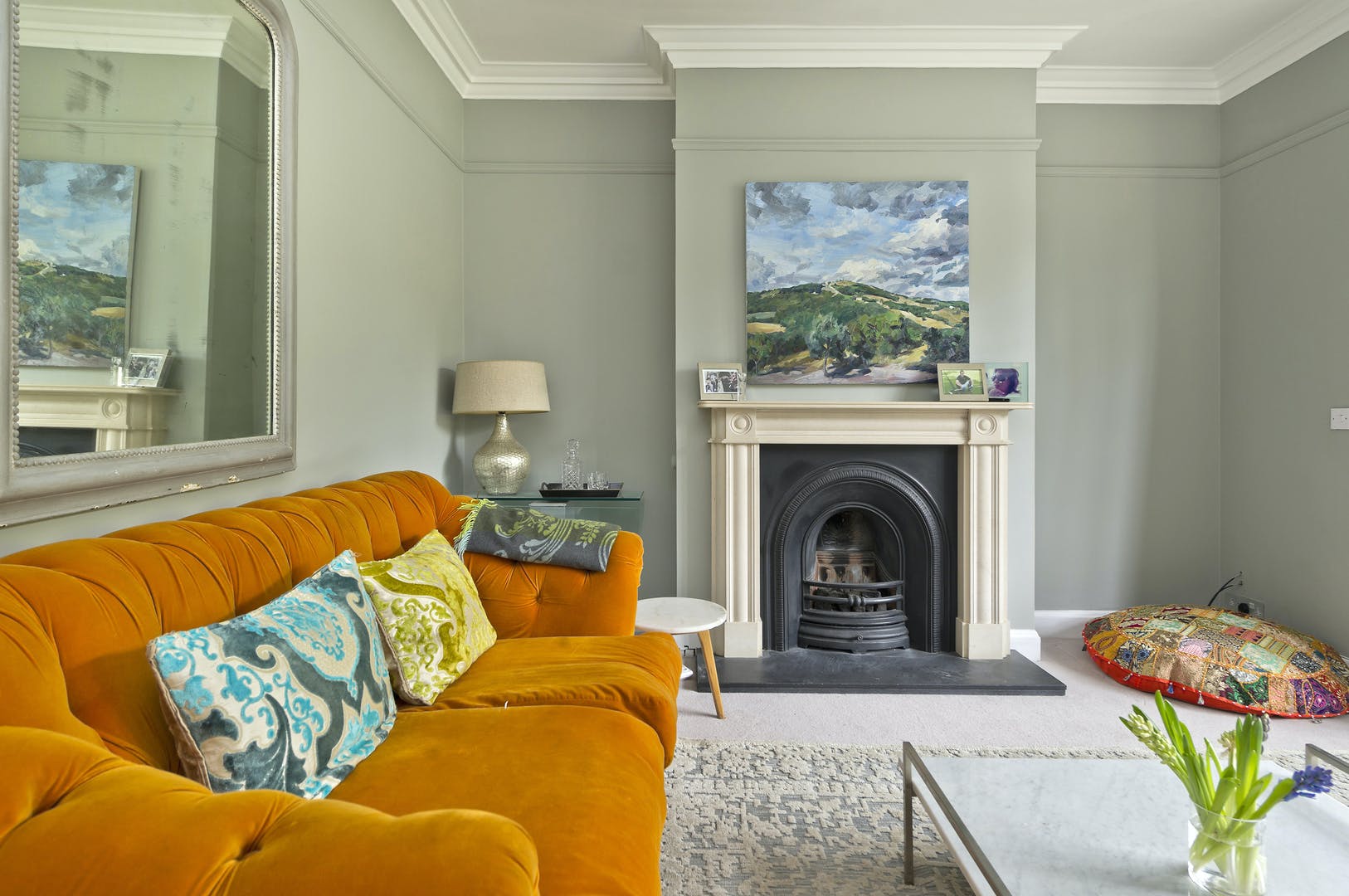In the living room, a plush and vibrant orange couch with decorative pillows in blue and yellow, each adorned with a fleur-de-lis pattern, sits prominently on the left-hand side. Above the couch hangs a mirror that reflects a fireplace at the opposite end of the room. The fireplace features an arched design and holds a metal pot filled with artificial logs or coal, its edges trimmed in a classical Caesarean style with white columns featuring indents for added texture. On the mantle of the fireplace, three photo frames are arranged, and above it, a painting depicts a mountain landscape with a grassy field. The room itself is characterized by light gray walls and matching carpet, with a white ceiling adorned with trim. The coffee table is white with gray trimmings, holding a plant, which complements the cozy yet elegant ambiance. Other elements in the room include a blanket draped over the arm of the couch, a floor cushion, a lamp, and what appears to be a bar cart.